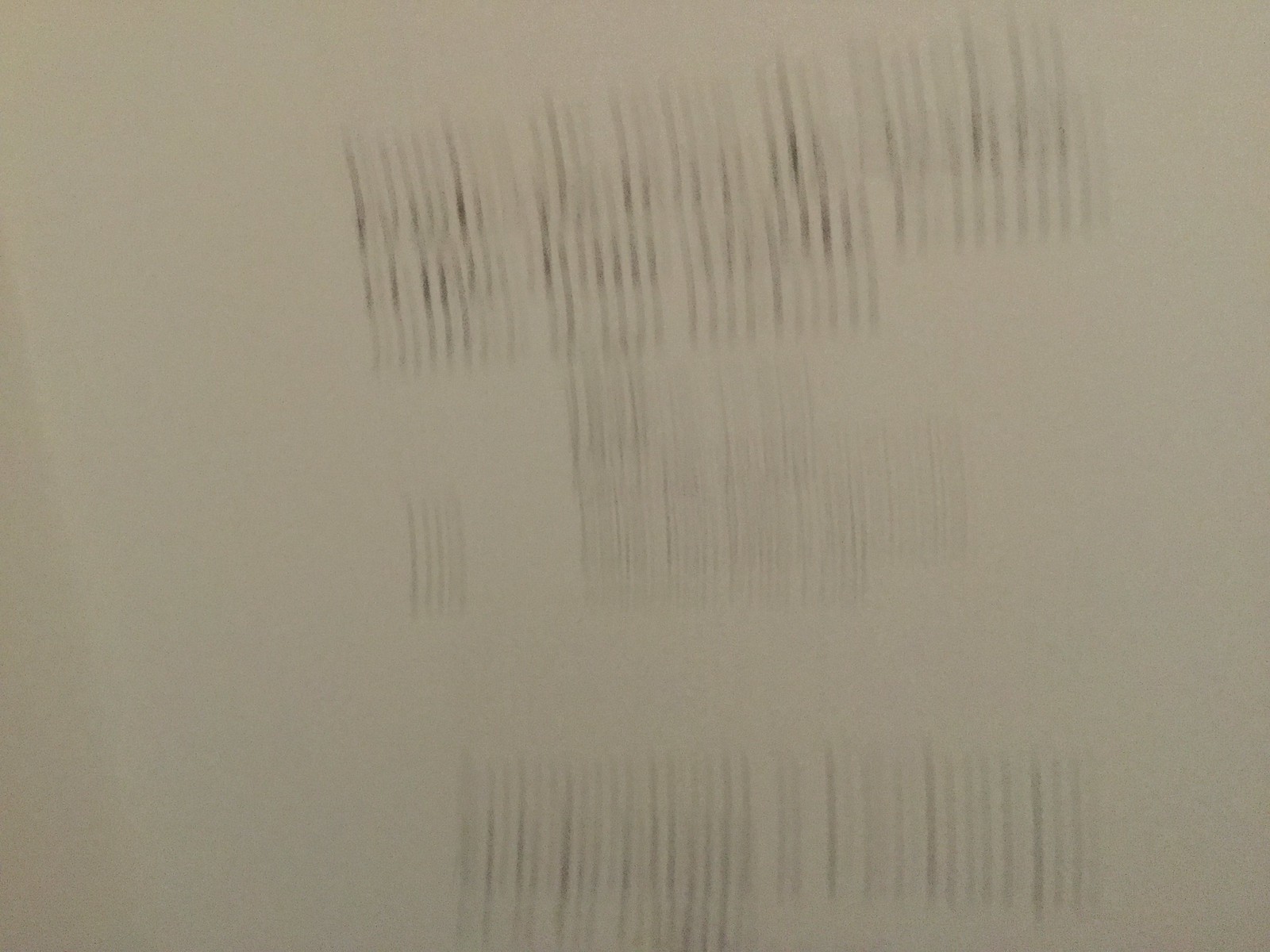The image depicts what appears to be black text on a white sheet of paper, rendered almost indecipherable due to rapid motion, resulting in significant blurriness. The characters have been stretched into elongated, vertical lines, making it difficult to distinguish whether they are letters or numbers. The top portion of the image seems to contain three rows of text that have been smeared into streaks. The middle section shows one or two rows of finer print, in comparison, appearing slightly less distorted but still largely unreadable. The bottom portion presents another one to two rows of text, which are not as fine as the middle ones, yet not as bold as those in the top section.